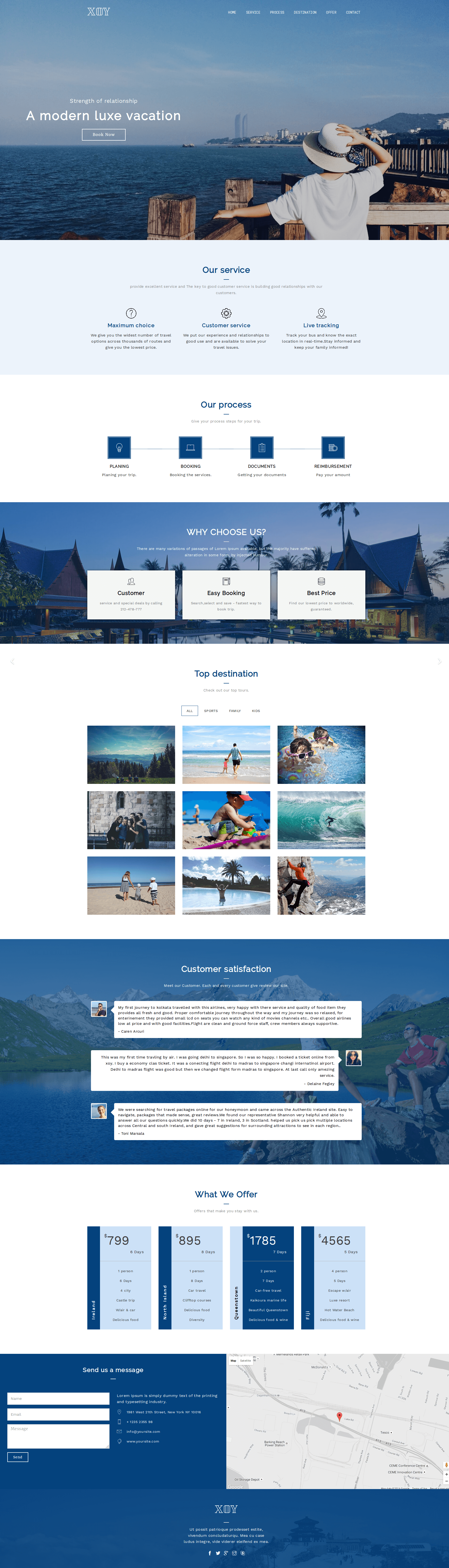The webpage features a detailed travel-themed layout, albeit the initial image appearing very zoomed-out and small. At the top, located on what seems to be the navigation bar, is a blurry image which shows an individual standing beside a road or pier, bordered by a metal barrier supported by wooden posts. The person, viewed from behind, is dressed in a white T-shirt and white hat, with their right hand holding onto their hat as the sun shines behind them. The background reveals a vast blue ocean, portions of land with mountains, some buildings, and a mix of gray clouds interspersed with patches of blue sky. Superimposed white text on this image reads "A Modern Luxe Vacation," with additional illegible options in white at the top.

Beneath this image lies a lighter blue section featuring blue text and three black text sub-menus, followed by a white section containing possibly four blue-tinted screens or options. Directly below this is another image depicting bungalows with distinctive, pointed roofs reminiscent of Thai architecture, surrounded by palm trees at what appears to be sunset or early sunrise, illuminated by the bungalow lights.

Further down, a section titled "Top Searches" displays nine images arranged in three rows. The first row includes an image of a forest, a beach scene, and two people swimming in a body of water. The second row features a grand building, a group of people on a beach, and a surfer. The last row shows three individuals walking on a beach, a person in clear blue water near palm trees, and a climber scaling a mountain.

Towards the bottom, a blue box likely contains reviews, showcasing three comments each with a white avatar box and black text. The faint background shows a person in an orange shirt and shorts seated on rocky terrain beside water and mountains. Lastly, the lower segment of the page consists of four blue informational boxes, and a predominantly blue section designed for personal information input, adjacent to a gray map with an orange arrow. The footer includes white text against the blue background.